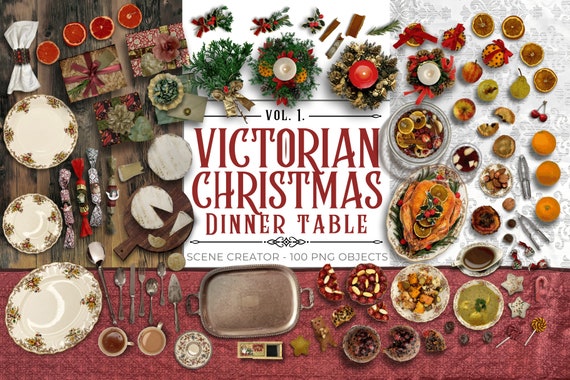A detailed top-down view of a Victorian Christmas dinner table, designed as a scene creator with 100 PNG objects. In the middle of the image, a white banner reads "Volume 1 Victorian Christmas Dinner Table. Scene Creator. 100 PNG Objects." Surrounding this central text are various elements featuring a luxurious holiday feast. 

In the top left, a segment of a wooden table is visible, while to the right, there’s a plush brocade table. The scene includes a vibrant red tablecloth adorned with an assortment of festive items such as presents and evergreen decorations with bows. Centerpieces featuring pinecones, branches, and flowers are interspersed among the dishes.

A delicious array of food dominates the table, featuring a roasted turkey, an apple tart, a half-eaten mincemeat pie, and a variety of fruits including oranges and apples. Stuffing, lemon wedges, nuts in a nutcracker, and raisins complete the edible ensemble. Cheese logs wrapped in decorative cellophane harken back to gift baskets from the 80s and 90s. There are also old plates, silver platters, a cutting board with cheese, and a gravy boat filled with gravy. Dishes, coffee cups, and intricate utensils add to the ornate setup, making the scene a rich tapestry of Victorian holiday dining.

The objects stand out against various backgrounds, some with drop shadows to enhance their realistic placement, indicating the collection’s purpose as a versatile and comprehensive design resource.